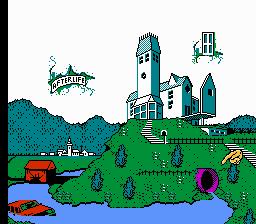This square-format, computer-generated, 2D cartoonish image depicts a whimsical scene centered around a green hill with a white building or house featuring bluish-colored, sloped roof areas. At the hill's summit, the structure includes a large steeple or tower, adding to its distinctive appearance. Surrounding the property is a blue lagoon, akin to a half moat, in which a red car is peculiarly half-buried or floating. In the foreground, towards the bottom right of the image, an unusual rabbit can be spotted. The upper left-hand corner of the image displays the word "afterlife" encircled by green, crack-like designs, suggesting a fantastical or video game-like environment. Adding to the surreal atmosphere, a purple tube protrudes from the side of the green hill, and distant mountains frame the background of this imaginative landscape.